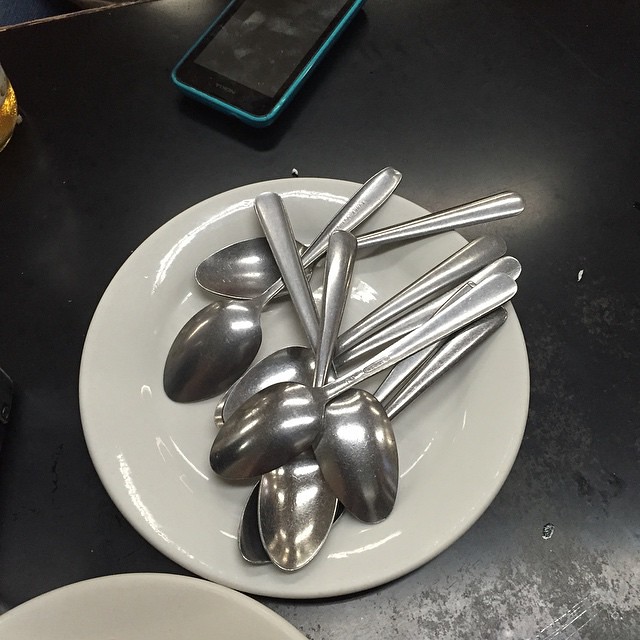This image captures a minimalist interior scene centered around a reflective, black countertop or table. In the middle of the image, there's a well-lit, medium-sized white plate, positioned just below the center. The plate, which seems to glow under the overhead light, holds a scattered pile of polished silver spoons, totaling around seven or eight, with their handles generally facing the same direction, between nine o'clock and six o'clock. The spoons overlap randomly, adding to the casual arrangement. In the bottom left corner, a sliver of another white plate is visible, adding depth to the scene. Towards the top center, a cell phone with a teal or turquoise blue case intrudes into the frame, tilted towards the seven o'clock position, suggesting an iPhone by the speaker hole visible. On the left side, partially obscured, is a translucent yellow object possibly a glass of juice or another beverage, through which light subtly filters, contributing to the overall reflective quality of the composition. The table itself shows a few smudges and signs of wear, adding texture to the otherwise clean and simple arrangement.